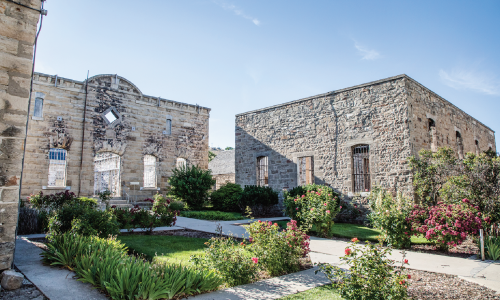The image depicts a sunlit courtyard framed by three ancient, rustic buildings made of light-colored, sandy stone that evoke a sense of old-world charm reminiscent of either Spain, Italy, or a historic western town. The courtyard is bordered by a stone sidewalk that leads to the entrances of each structure. On the left, the building is mostly obscured, with only its corner visible. The central building, slightly set back, features an arched doorway with a diamond-shaped window above it; its windows bear white bars and it might be roofless. To the right, the square building also appears to be without a roof and has brown bars on its windows. The well-maintained garden in the center is filled with lush greenery, vibrant flowers including striking red and orange blooms, as well as a prominent bush adorned with a multitude of pink flowers. The detailed stone and cobblestone structures, along with the bars on the windows, suggest a preserved historical site, possibly used for tours, akin to the Alamo in San Antonio, Texas.